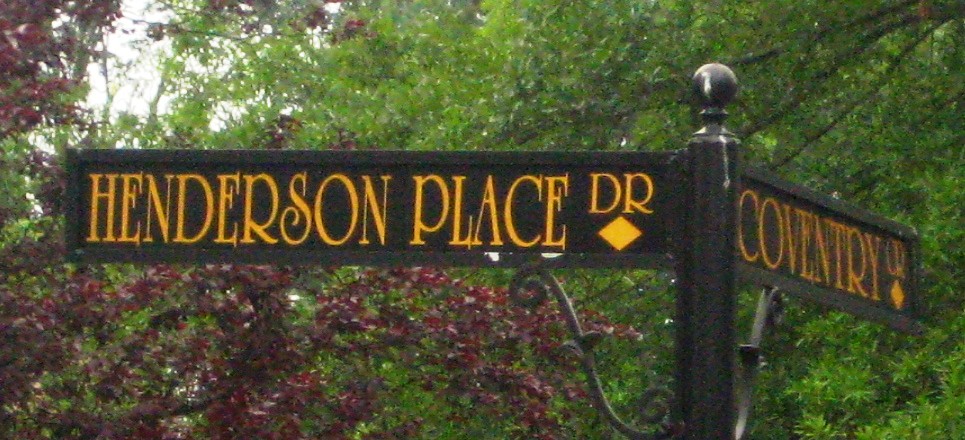A black street sign post, topped with a round black finial, stands prominently against a backdrop of trees. The sign features two arms extending at right angles to one another. Both arms are black with large, yellow capital letters. The left arm reads "HENDERSON PLACE DR," accompanied by a yellow diamond underneath. The right arm reads "COUNTRY DRIVE," also with a yellow diamond beneath it. The trees in the background exhibit a mix of green and copper hues, providing a picturesque and natural setting. In the upper left corner of the image, a glimpse of the sky peeks through the foliage.